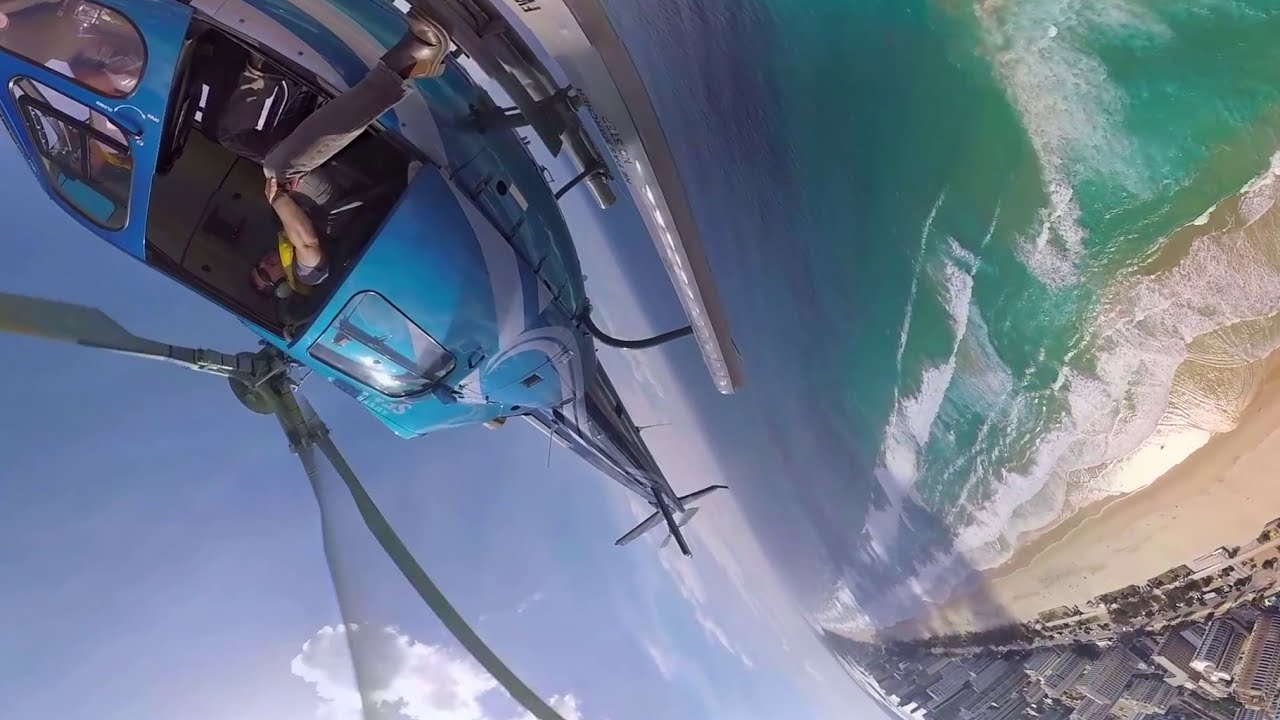The photograph captures a dynamic aerial perspective, as if taken from a slightly tilted angle, emphasizing the scenery below. At the forefront, a blue helicopter with white stripes on its hull hovers above a pristine beach. The helicopter's side door is open, revealing a relaxed individual sitting with a black sunglasses, confidently resting their leg on the helicopter skids. The helicopter blades, seen in a blurred motion, are a gray color.

Below, the beach unfolds in a serene tan hue, untouched by any beach-goers, alongside a ribbon of aquamarine water close to the shore that deepens into a darker blue further out. Waves crash against the shore, their foamy white crests visible amidst the vibrant blue-green waters. To the side, a line of houses stretches along a two-lane road, marking the boundary between human habitation and the natural beauty of the beach. The sky, predominantly clear with just a few wispy clouds, adds a touch of blue to the left side of the image, framing the scene in a bright, sunny day. The overall tilted perspective contributes to the dynamic and somewhat disorienting feel of the photo, accentuating the breathtaking aerial view.